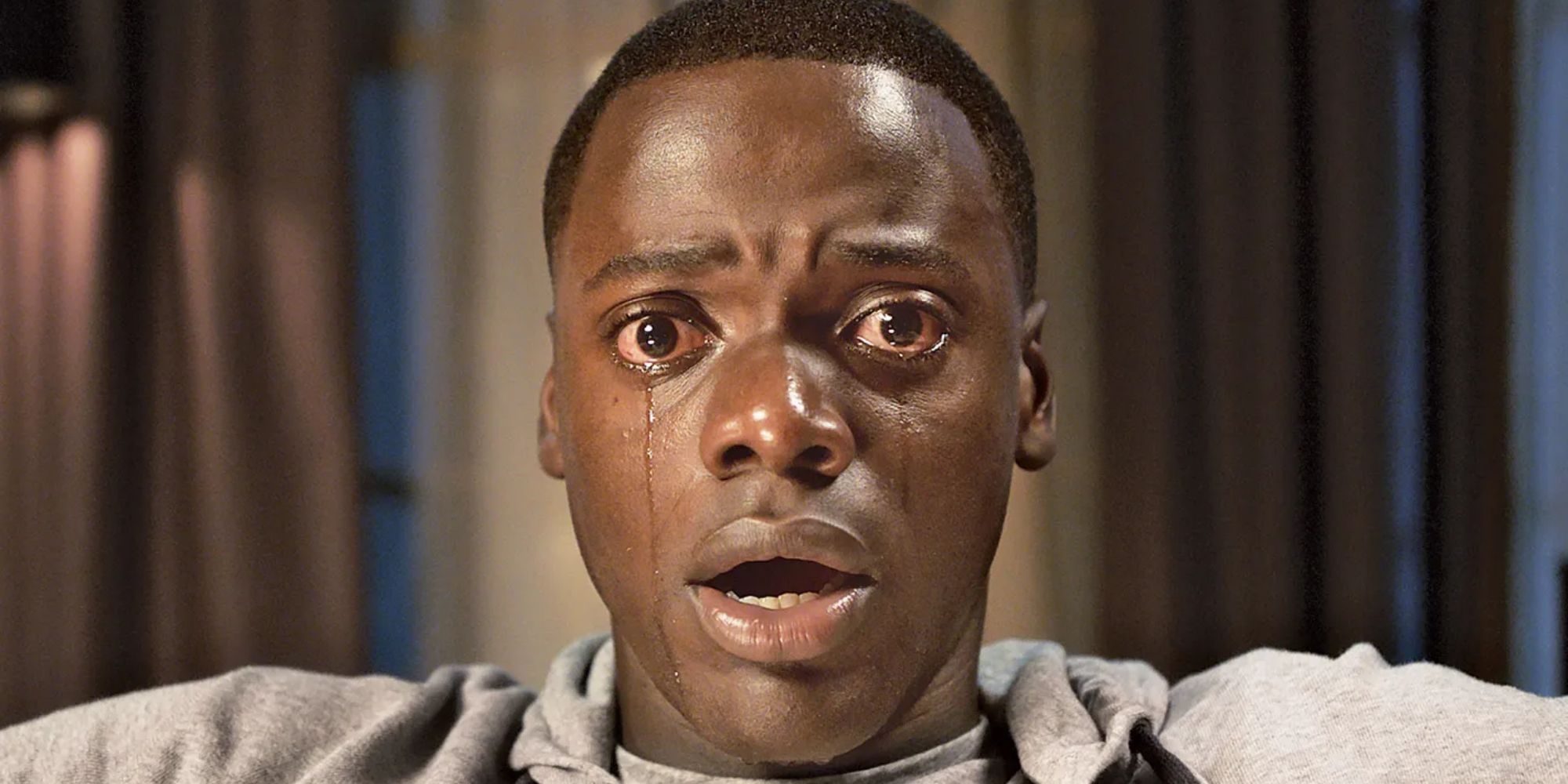The image depicts a young black man, approximately 17 or 18 years old, sitting down and looking straight ahead with a gaze of astonishment and shock. He has short-cropped hair and is wearing a light gray hoodie over a gray t-shirt. His eyes are visibly red and bloodshot, indicating he has been crying for some time, with tears streaming down his face—one tear especially prominent on his right side, extending down below his mouth, and another tear on his left side, reaching the center of his cheek. His forehead is tensed, eyebrows drawn inward, and his mouth is moderately open, revealing his lower jaw and teeth. His nostrils are also flared, adding to his expression of surprise. The background consists of brown curtains flanking either side, partially covering a beige wall and a window. The setting is softly lit, accentuating the emotional weight of the moment captured in this digital screenshot.